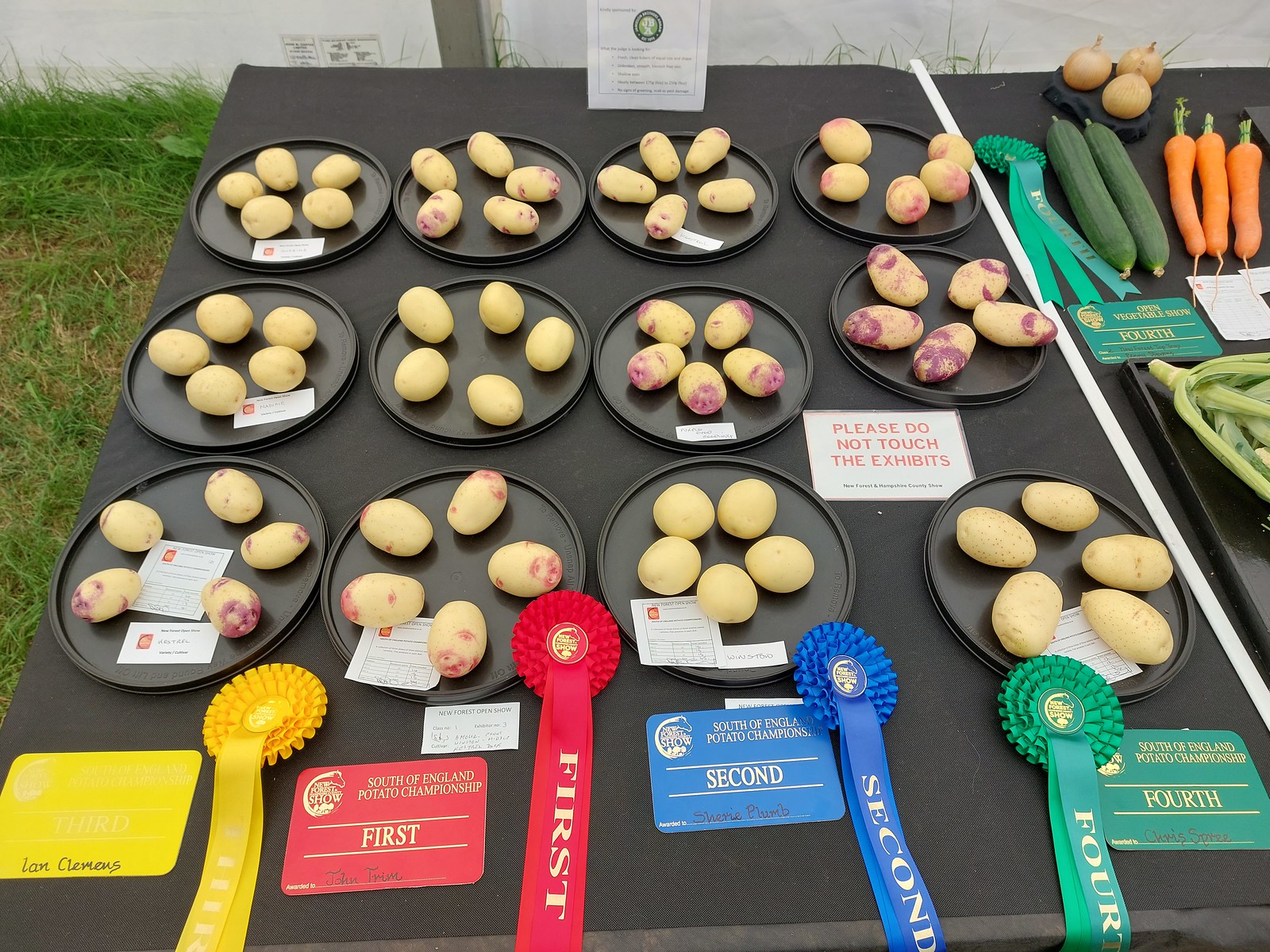In the image, there is a large black table covered with a black drape, positioned on a grassy area. A white stripe runs down the middle, giving it the appearance of a ping-pong table. Neatly arranged on the table are 12 black plates, each encircling five peeled potatoes. The potatoes vary in appearance, with some being white and others displaying purplish or pinkish hues. A sign on the left side of the table reads, "Please do not touch the exhibits." This table seems to be part of a potato contest, as evidenced by ribbons placed on the plates: a yellow ribbon for third place on the far left, a red ribbon for first place next to it, a blue ribbon for second place further right, and a green ribbon for fourth place on the far right. Beside the main table, to the upper right in the image, there is another black table holding an assortment of vegetables like cucumbers, carrots, and onions, along with a sign stating "South of England Potato Championship" and a plaque for the "Fourth Open Vegetable Show."